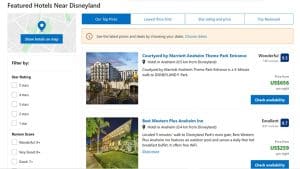The image depicts a webpage for finding hotels near Disneyland. In the middle of the webpage, there is a small, difficult-to-read map with a pin indicating the location of Disneyland hotels. Below the map, there is a list of two hotels. Each hotel listing includes the name of the hotel, such as the Courtyard, and a star rating on the right. The price of the hotel is displayed in green text, and there is a blue button that reads "Check Availability." Additionally, there is a "thumb" icon, presumably for user reviews.

The second hotel listing shows a price around $230 and includes the word "excellent," indicating a high rating, but the hotel's name is not legible.

On the left-hand column, under the map pin, there are filtering options. You can filter hotels by star ratings (one, two, three, and four stars) and other features, though the specific amenities are not entirely readable. It suggests options to filter by the number of bedrooms, bathrooms, and possibly amenities like spas.

At the top-right section of the page, there are four boxes for different options, with the currently selected one highlighted in blue. Below these boxes, there seems to be a disclaimer, but the text is unreadable.